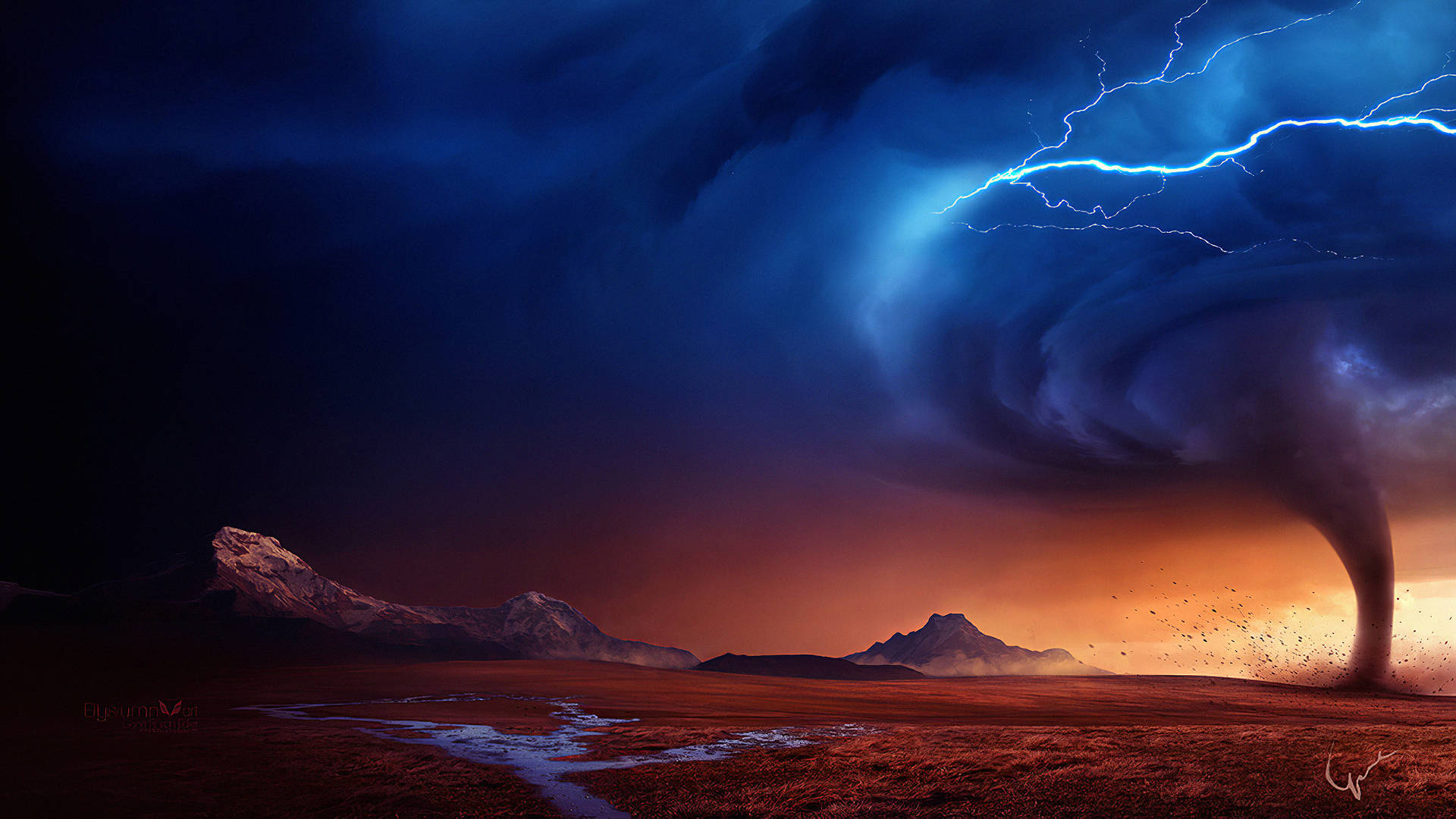This captivating painting depicts a dramatic scene of a ferocious tornado sweeping across a rugged landscape. On the right side of the image, the tornado's funnel stretches from the ground to the sky, transitioning from a rust color at the base to a darker blue towards the top. The tornado’s chaotic energy is evident, with debris and dust swirling around its base.

Above, the sky is a mesmerizing gradient, shifting from dark blue at the top to lighter blue closer to the enormous funnel cloud. Surrounding the tornado are ominous dark clouds, almost black towards the left, punctuated by a striking lightning bolt branching from the left side of the funnel. The horizon is bathed in orange and yellow hues, contrasting starkly with the darker stormy sky.

The landscape beneath the tumultuous sky features an orange ground, with a small stream or brook flowing on the bottom left. On the horizon, small mountain peaks rise, with a larger mountain in the center left and a hill on the far left. In the bottom right-hand corner, an antler logo subtly marks the canvas, adding a unique touch to this intensely atmospheric scene.